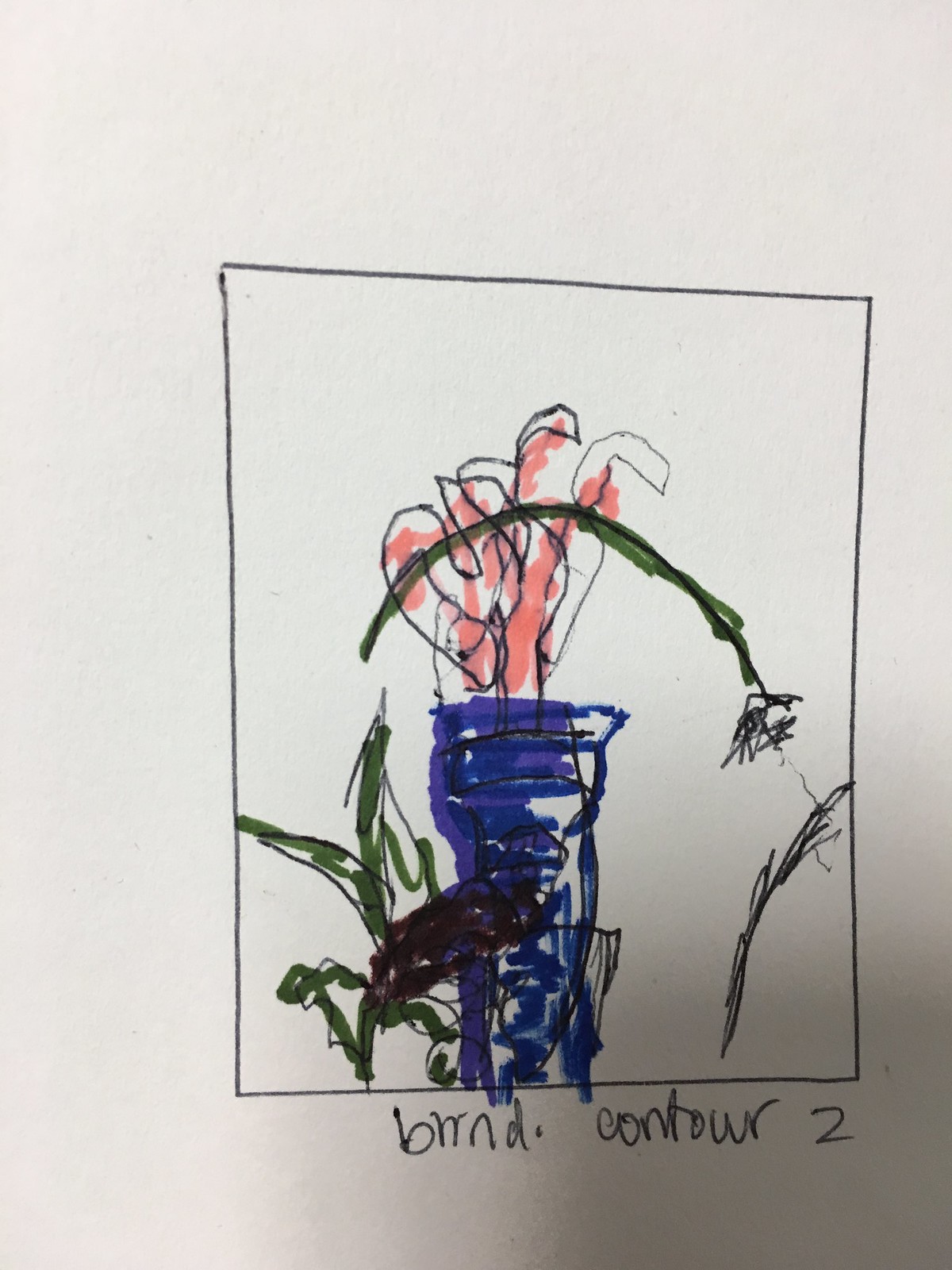The image appears to be a photograph of a hand-drawn or hand-painted artwork. Central to the composition is a black square, within which an abstract representation of a hand is depicted. Starting from the elbow, a blue line extends up to the wrist, transitioning into the hand itself, which is portrayed with sinuous, snake-like forms and shaded in a reddish-pink, skin-like tone.

The hand is shown grasping a green stem that leads to a flower. The flower is intricately sketched with delicate black lines, from which a solitary black line seems to fall. On the left side of the image, sharp green lines are also visible, adding to the abstract nature of the piece. Below the black square, the text "brnd.contour2" is inscribed, hinting at the possible title or series name of the artwork.